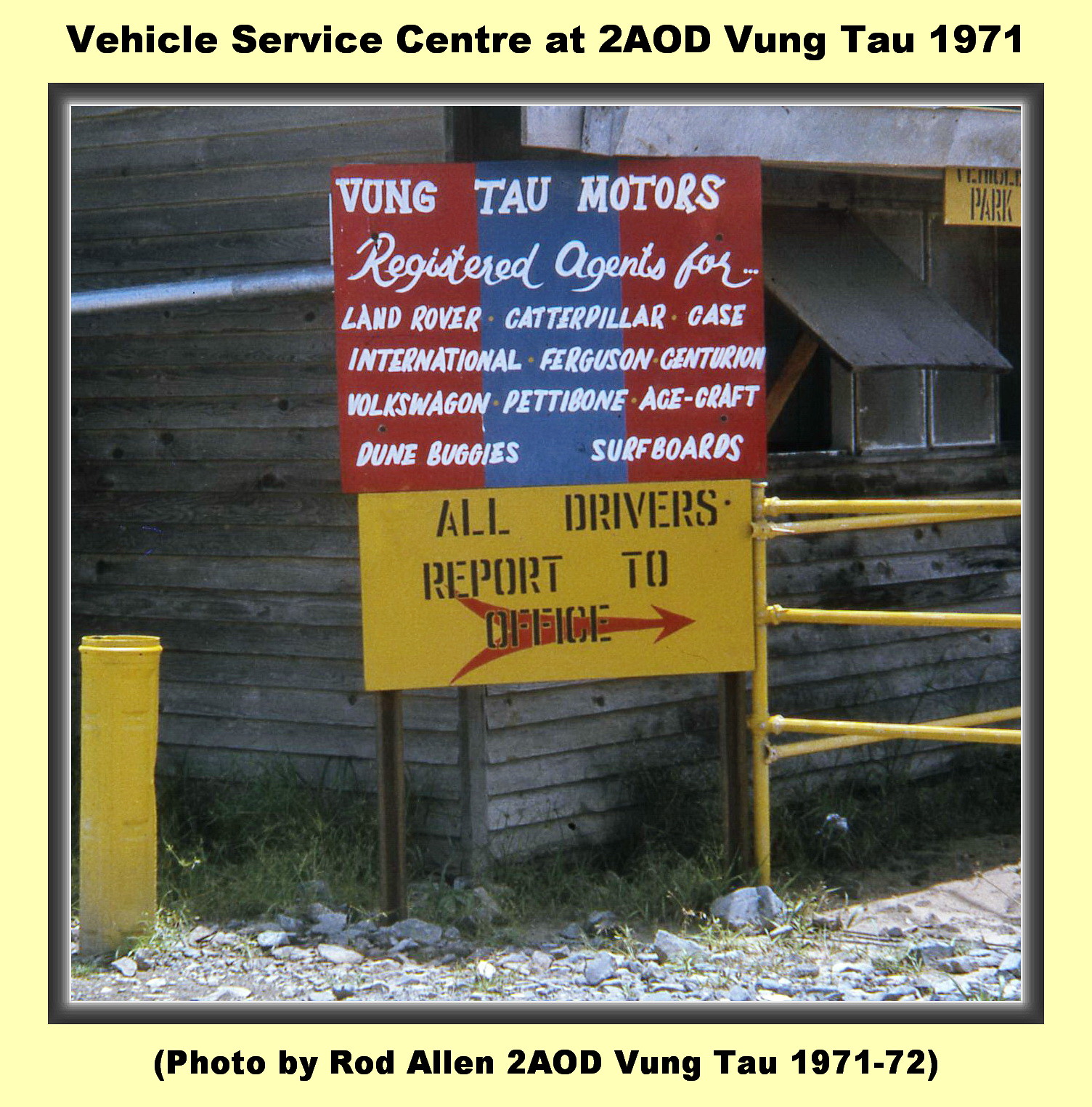This detailed photograph captures an outdoor scene featuring a vibrant sign in front of a corner of a wood building. The sign itself is a colorful mosaic with red, blue, and yellow sections and displays text in black and white letters. The top portion of the sign reads "Vumtau Motors," identifying registered agents for brands such as Land Rover, Caterpillar, Case, International, Ferguson, Centurion, Volkswagen, Pettibone, Age, Craft, Dune Buggies, and Surfboards. This text is set against vertical sections of red, blue, and then red color blocks. The lower part of the sign, in black letters on a yellow background, instructs "All drivers report to office," with a red arrow pointing to the right.

In the backdrop, the wood building shows a window toward the right side. Towards the bottom right, in front of the building, there's a yellow fence, likely made of metal rods. The photograph is bordered in light beige, with the top indicating "Vehicle Service Center at 2AOD Vumtau 1971," and the bottom crediting "Photo by Rod Allen 2AOD Vumtau 1971-72."